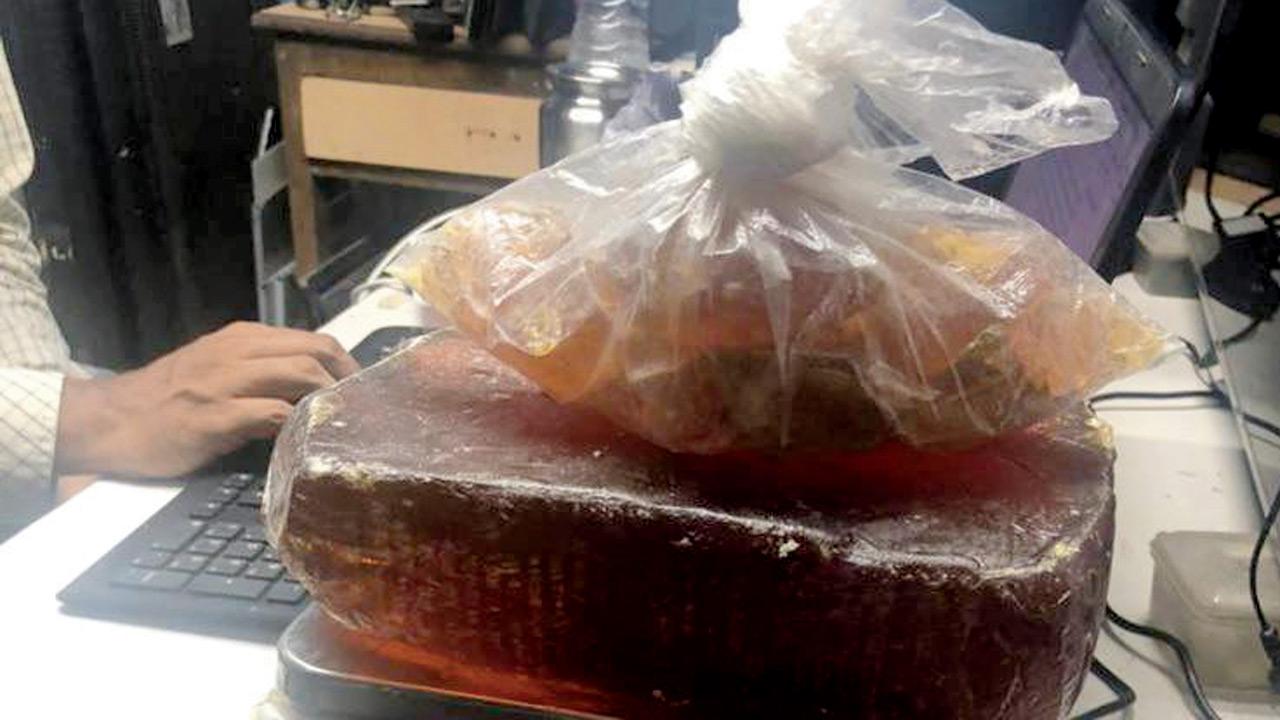In a brightly lit, overexposed color photo, a man's hand, clad in a white checkered long-sleeved shirt, is visible as he types on a black laptop keyboard. To the right of the keyboard sits a silver boxy scale, possibly connected to the laptop by wires. On the scale rests a large, amber-colored, translucent irregular block, wrapped in a plastic covering. Atop the block is a clear plastic bag, knotted and filled with what appears to be chunks of a similarly waxy or candied substance resembling orange and lime peels. The scene is set against a backdrop featuring a white-cluttered table and a wooden nightstand with visible drawers. The man seems to be in the process of weighing the items on the scale, indicating a setting that could be either domestic or related to some form of manufacturing or evidence processing.